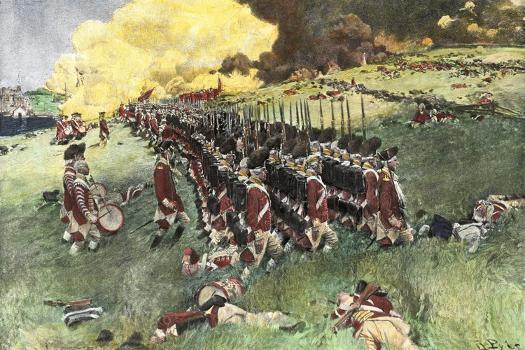This detailed painting depicts a Civil War battle scene in a landscape layout, spanning from the bottom left to the top right. The central focus is on three rows of 18th-century soldiers dressed in red coats and white, sometimes beige, pants. They wear large black hats and carry rifles pointed upwards on their shoulders. These soldiers are marching upward on a grassy incline, with a few men trailing behind, including one carrying a drum.

Scattered across the grassy field, which is depicted with tall grass, are casualties in identical uniforms, indicating the brutality of the battle. In the background, a significant cloud of white and yellow smoke merges with darker, blackish-brown smoke, adding to the chaotic atmosphere.

Further details include stone walls in the field and a building visible in the upper left corner, set against a grayish-blue sky. The soldiers are organized, advancing rightwards across the inclined landscape, towards more fallen comrades visible in the distance amidst the smoky and turbulent background. This painting vividly captures the confusion and intensity of a historical military encounter.